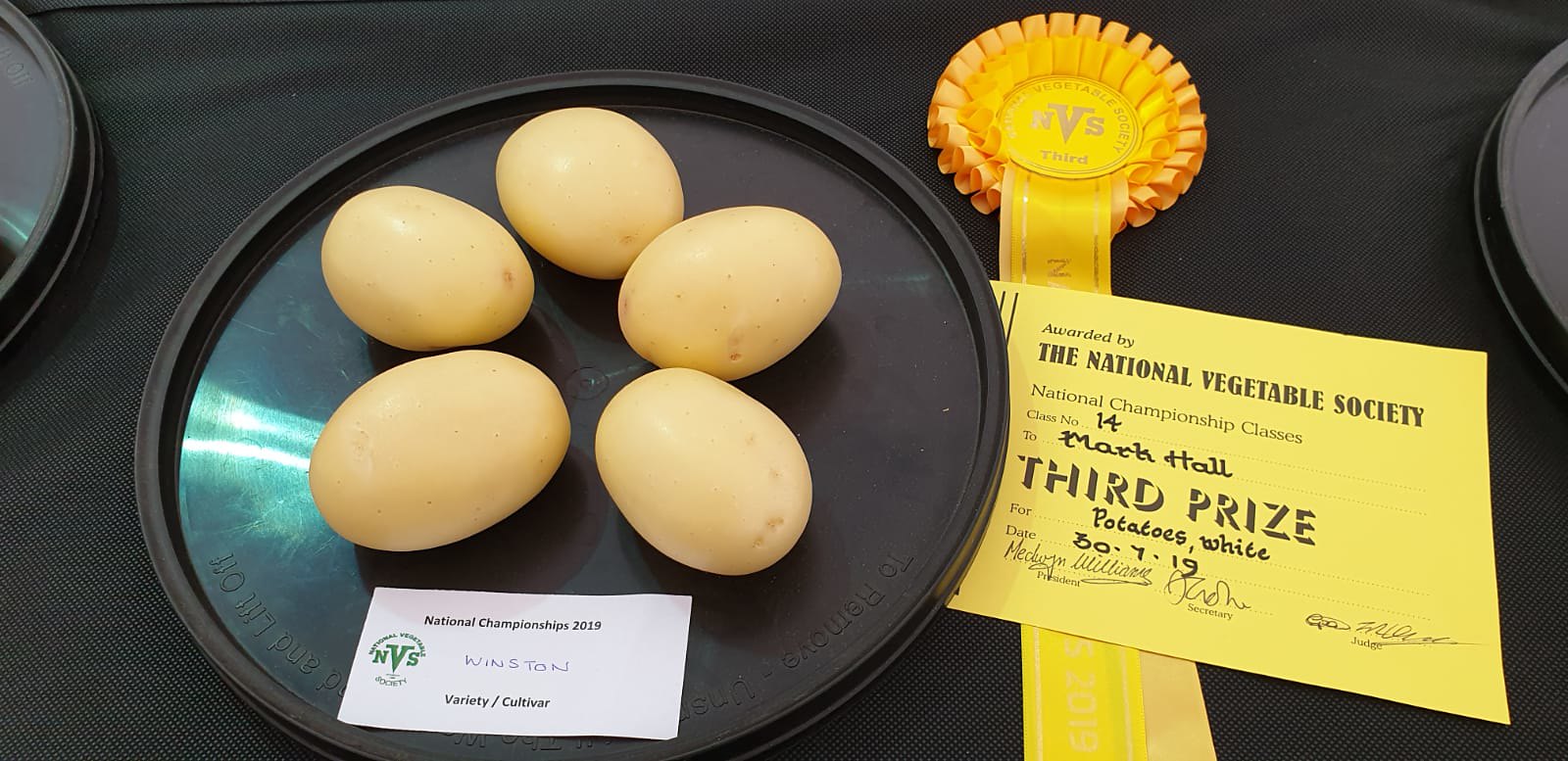The image depicts five smooth, white potatoes arranged in a circular pattern on a black plate, positioned at an agricultural competition. The potatoes have been awarded third prize by the National Vegetable Society in the National Championship Classes, Class No. 14, for the cultivar (or variety) 'Winston'. A yellow ribbon is prominently displayed next to the plate, featuring a certificate that reads "awarded by the National Vegetable Society, National Championship Classes, to Marla Hall, third prize, potatoes, white," dated July 30, 2019, with several signatures underneath. The plate also has a small sticker indicating "National Championships 2019 Variety/Cultivar," confirming its participation and recognition. The setup rests on a black cloth, surrounded by the edges of nearby trays visible on the left and right.